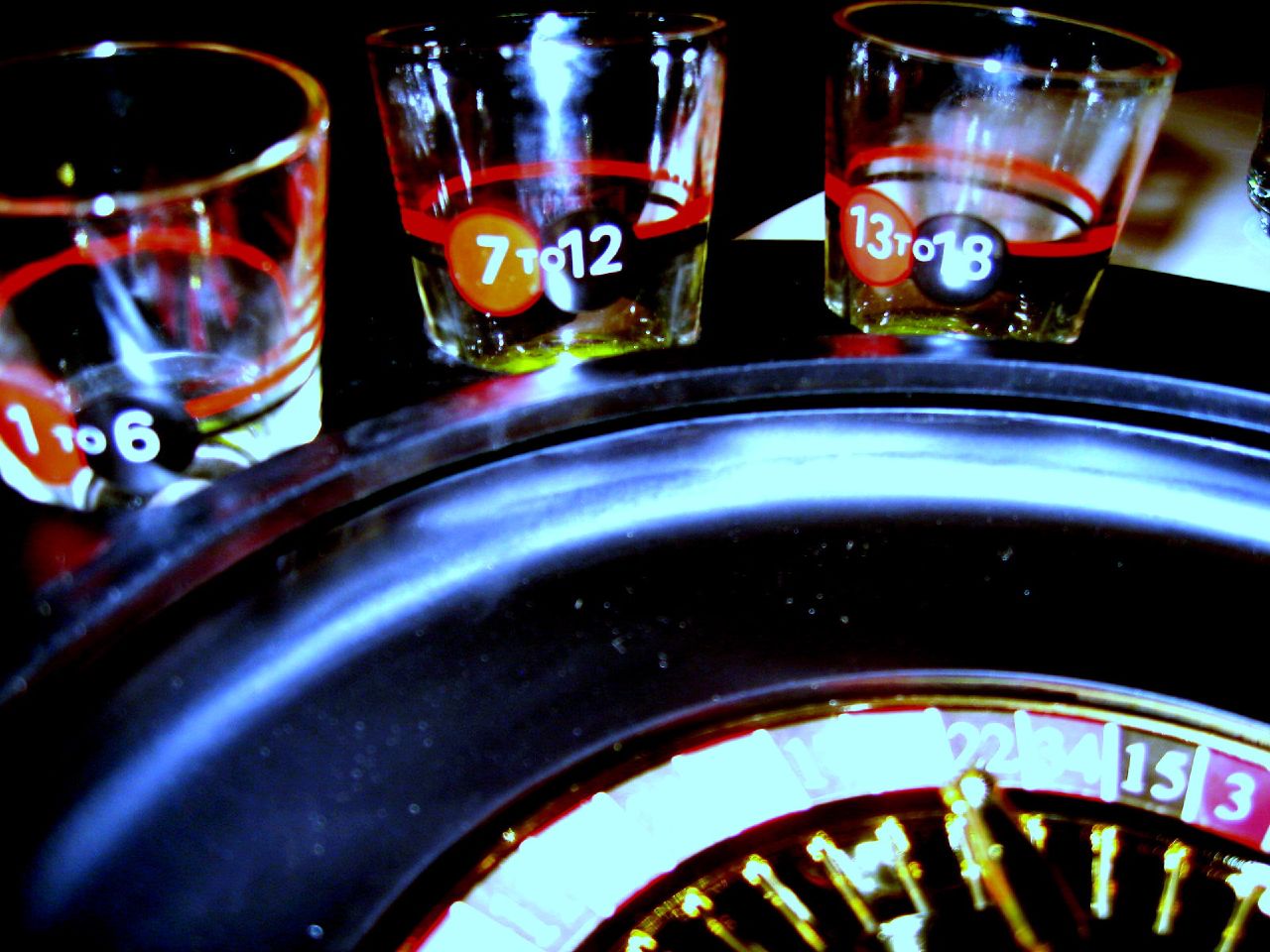This image features an extreme close-up of a roulette wheel, appearing prominently in the lower right corner, with only part of the wheel visible due to overexposure from the camera flash. The identifiable numbers on the wheel include twenty-two, thirty-four, fifteen, and three. The roulette wheel exhibits the classic red and black numbered spaces and is accented with a silver-and-blue outer surface that curves elegantly.

In the upper portion of the image, set against a somewhat dark background, three clear shot glasses are arranged as part of a drinking game set. Each glass is delineated with a prominent red line halfway up, reminiscent of a measuring cup, as well as smaller red horizontal lines. They feature white number ranges: the one on the left reads 1 to 6, the middle one displays 7 to 12, and the one on the right shows 13 to 18. Additionally, each number range is marked with circles under the numbers; red circles underneath the first number in each range and black circles beneath the second number. The shot glasses rest on what appears to be a white table, suggesting they might be involved in the betting aspect of the game.

The overall scene combines elements of a traditional casino roulette setup with an inventive twist, implying the addition of a drinking game.